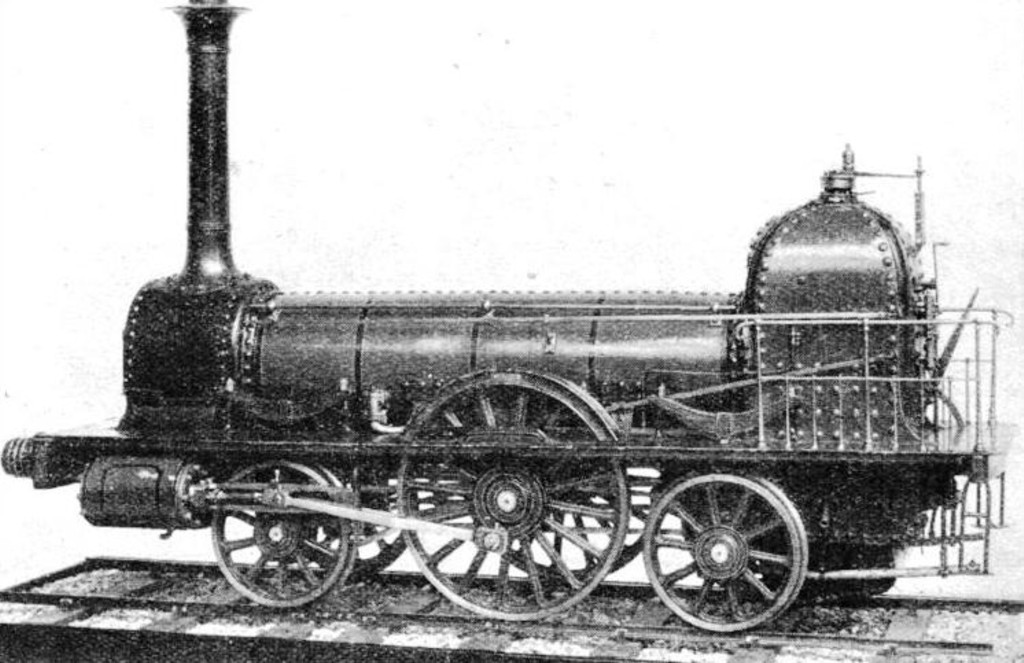This black and white photograph depicts a detailed model of a 19th or early 20th-century steam train. The train is oriented from a side view, with the front facing left and the rear to the right. At the front, a large smokestack extends upwards, indicative of its steam engine functionality. The main body of the train features a long cylindrical central section adorned with numerous metal rivets. Notably, the train sports three wheels: two smaller ones on either end and a prominent, large central wheel. The large wheel is connected by a metal bar to a piston situated beneath the smokestack, aiding in the engine's propulsion.

Towards the back, instead of the typical windows and cabin for an engineer, there is a tall, domed metal area, suggesting this model may have unique or incomplete elements. The entire assembly rests on a miniature train track, which sits on a black base with contrasting white sections between the rails. The photograph's white background contrasts sharply with the metallic gray, black, and white sheen of the train, enhancing the historical and mechanical details of this intricate steam engine model. A small metallic fence appears on the right side of the platform, adding to the scene's authenticity.